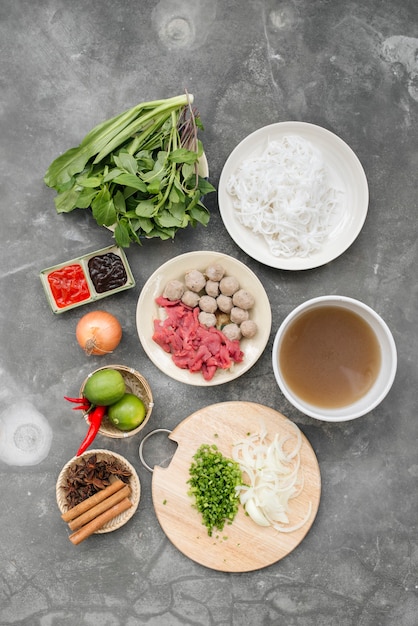In this overhead portrait-oriented photograph, the central focus is an array of cooking ingredients meticulously arranged on a gray, slate-textured background, rich with natural stone coloration and intricate cracks. At the top left of the image, a verdant bushel of green herbs or leafy vegetables contrasts brilliantly against the slate. Adjacent to this, a circular white plate displays fibrous white noodles or rice. Below these elements, a tin rectangle holds two types of sauces, one vibrant red and the other a deep brown.

Dominating the central area, an off-white plate presents an assortment of red meat pieces and possibly meatballs. Slightly below and to the right, a circular cutting board features finely chopped onions and green vegetables, potentially green onions. Enhancing this composition, a white bowl to the far right contains a clear broth. Scattered throughout are other culinary components, including bundles of onions, fresh limes, aromatic cinnamon sticks, red peppers, and an indication of the dishes' intended combination, likely contributing to a flavorful broth-based dish. This photograph exudes a minimalist yet modern aesthetic, highlighting the art of meal preparation.